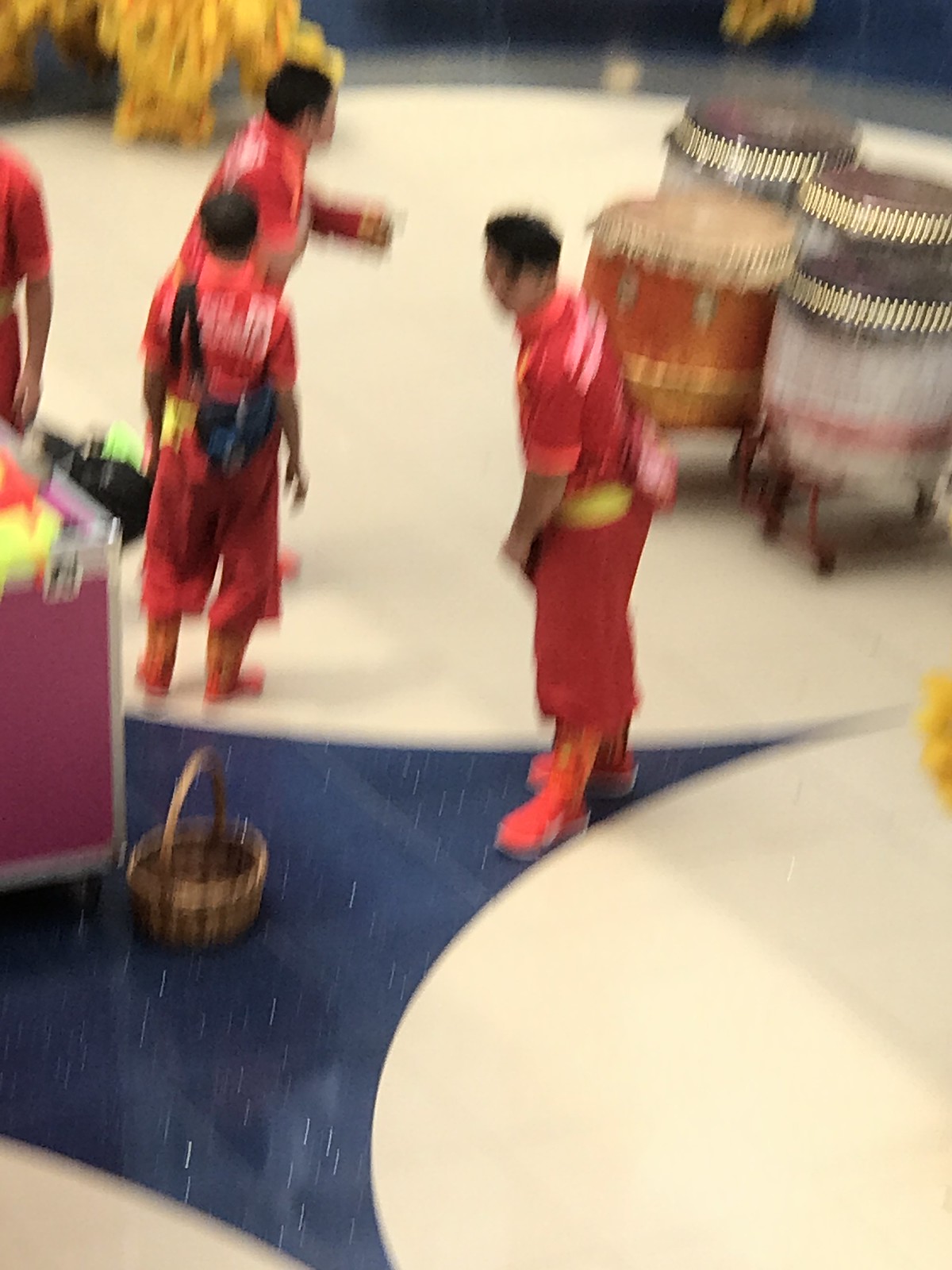The image captures a very blurry photograph of four young men with black hair, all dressed in bright red outfits adorned with white writing on the back. Each wears a bright yellow belt around their waist, and their pink and yellow boots are complemented by white soles. The men are stationed on a distinct white floor that features a blue star-shaped pattern at its center. Adjacent to the star lies a basket with a handle nestled on the ground and a pink wooden crate encased in a metal frame. In the background, four large bongo drums rest on small stands. One of the men is distinguished by a small black backpack. The overall scene appears to be an entertainment or practice venue where the figures seem engaged in carrying items from one place to another.